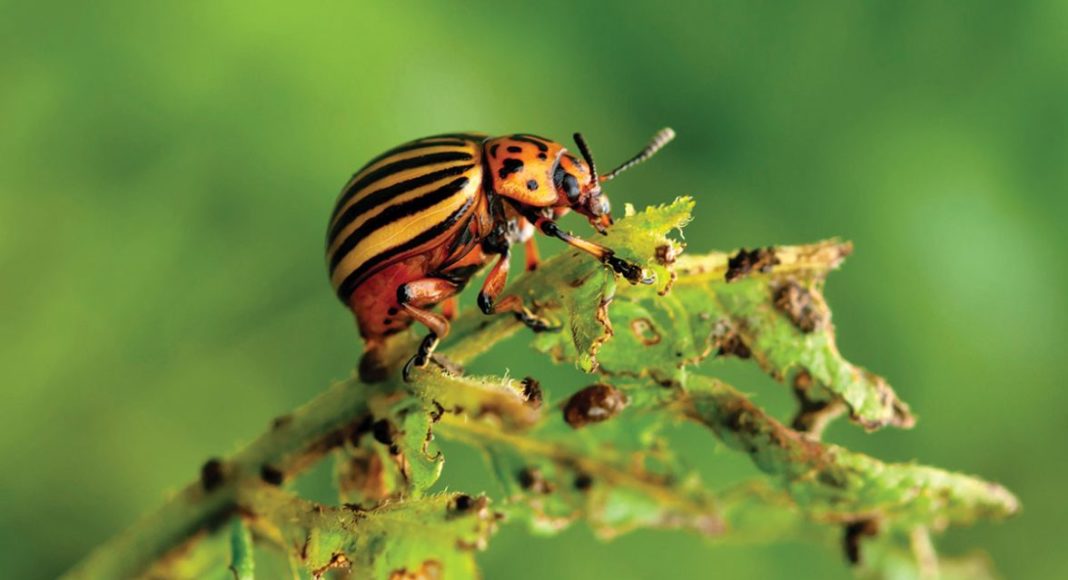This professional photograph showcases a close-up of a beetle perched on a plant stem with sickly leaves, possibly affected by mold. The beetle, reminiscent of a Colorado or potato beetle, displays vivid detail with a body comprising various intricate parts: a head that's black and brown, an orange and black-spotted thorax, and a hard, shell-like back adorned with yellow and black vertical stripes. The underside reveals reddish tones, while the legs are a mix of orange and black. Two distinct black and white antennae are prominent on its head. The background is blurred, featuring different shades of green, creating a strong depth of field effect that sharply contrasts with the crisp focus on the beetle and the stem. The stem itself, bearing numerous black spots, might be decaying. The image captures the beetle in the act of consuming the plant, with evidence of chewed leaves and possibly small piles of material around it, suggesting ongoing feeding.